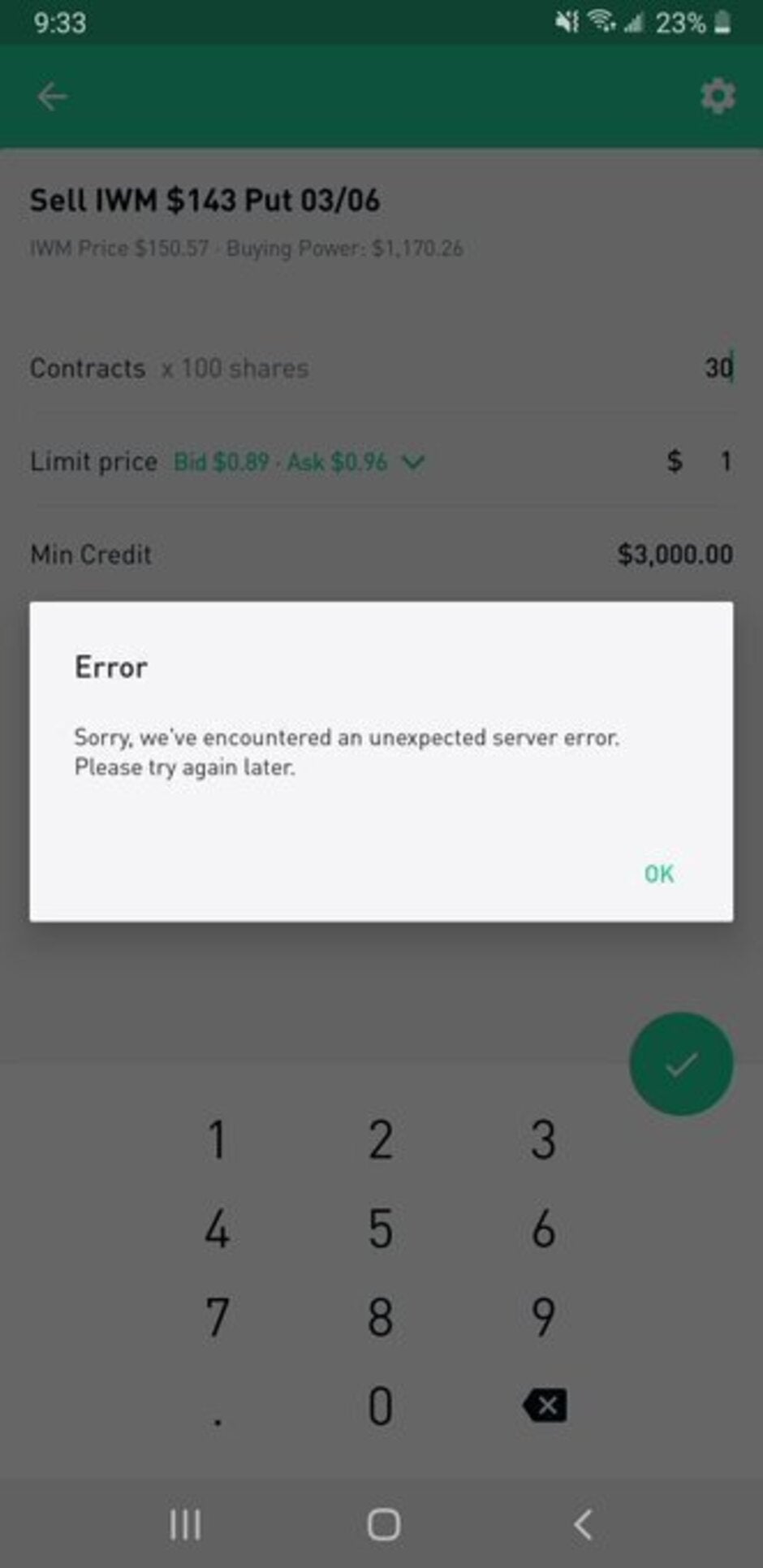The image is a screenshot taken on a phone, capturing an error message overlaying a dialing screen. The backdrop is slightly grayed out, revealing hints of a phone dialing interface. In the center of the screen, a white rectangular box displays a bold black header reading "Error" in a significantly larger font positioned at the top left of the box. Below this, the message, "Sorry, we've encountered an unexpected server error. Please try again," is centered within the box in smaller, black letters. At the bottom right corner of the error message box, a bright green "OK" button is visible, presumably for closing the error prompt.

Above this white box, the top part of the screen features a dark green bar with a white arrow on the left side, indicating a back navigation option. To the right of this bar, a small gear icon signifies the settings menu. Directly below this bar, in bold black letters, is the text: "Sell IWM $143.00 Put 03-06." Further down, also in bold black letters, it reads "IWM price $150.57, Buying power." This suggests the presence of a trading or financial application running in the background.